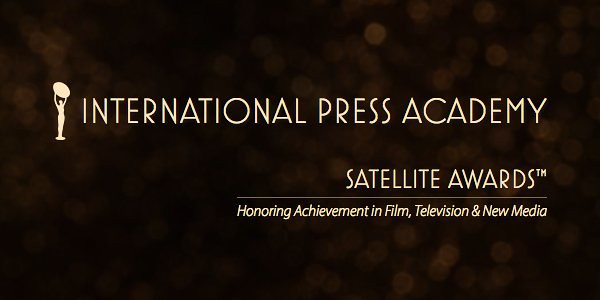The image serves as an advertisement for the International Press Academy's Satellite Awards, honoring achievements in film, television, and new media. It features a primarily dark, blurred background with a bokeh effect of soft, gold, and orange lights, creating an aesthetically pleasing yet unobtrusive backdrop. On the left side of the image is a goldish-white, faceless figure of a person holding up a round object, resembling a trophy, symbolizing the award. To the right of this figure is text in a corresponding goldish-white color, detailing "International Press Academy" in all caps, followed by "Satellite Awards™" and "Honoring Achievement in Film, Television, and New Media" in smaller, italicized sans-serif font. The entire composition effectively highlights the prestigious nature of the awards through its elegant use of color and layout.